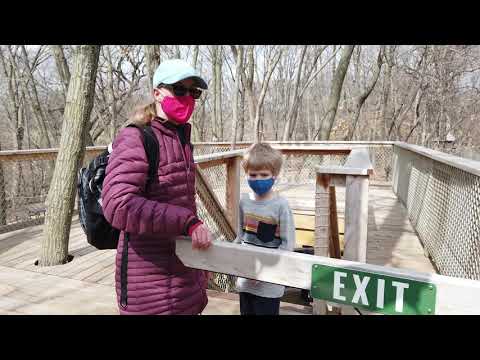In this detailed image, a tall female stands on the left side of an outdoor wooden platform, which features a tree growing through its center and a weather-beaten wooden lattice barrier. She is wearing a heavy purple coat, a blue cap, sunglasses, a pink mask, and a black backpack. She has one hand resting on a light yellow plank of wood that bears an exit sign with "Exit" written in white text on a green background. The person beside her, thought to be her son, is about half her height and has blonde hair, a blue mask, a gray shirt adorned with yellow, pink, red, and black stripes, a black patch, and black pants. They are surrounded by thick, leafless trees and dark, thick black lines cut across the screen, adding to the outdoor, possibly amusement-related setting suggested by the exit sign and the dock-like wooden platform.